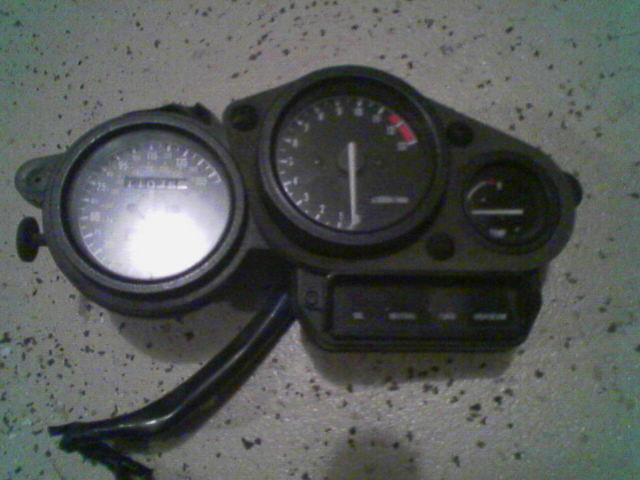This horizontal image, slightly wider than it is tall, features a distinct black object at its center, predominantly shaped like a triangle with a small rectangular extension in the lower right corner. This object comprises three gauges, each meticulously designed to convey critical measurements.

The largest gauge occupies the entire left side of the triangle. It appears to measure speed, akin to a speedometer, with numerical markers and a section dedicated to counting miles, reminiscent of an odometer in a car. The second gauge is positioned slightly above and to the right, forming the apex of the triangle. This gauge includes a red zone at the final 10% of its range, with a white needle and white numbers, though the exact measurement function is unclear. The final gauge, located in the lower right of the triangle, resembles a gas meter. Adjacent to this gauge, within the rectangular extension, are four indistinguishable words spaced apart, likely indicating alert lights without visible defined screens.

Emerging from the center of the object, angled towards the lower left corner of the image, is a tube, possibly a conduit for fluid or data. Overall, the intricate design and placement of these elements suggest a highly functional and specialized instrument panel.